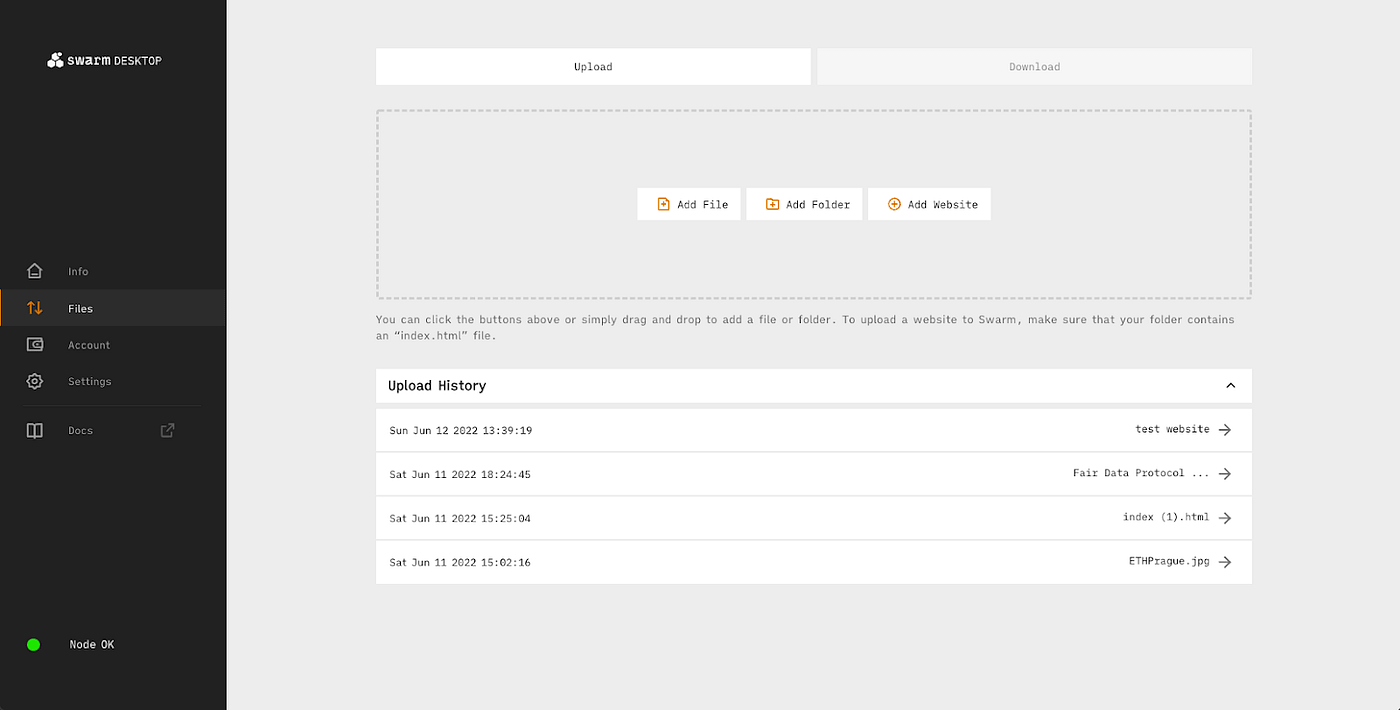This image is a screenshot of the backend interface of the Swarm Desktop application. The left side features a black sidebar with white text, with the application name "Swarm Desktop" prominently displayed at the top, albeit in slightly blurry text. The sidebar contains multiple buttons, each paired with an icon: a home icon next to "Info," an up and down arrow icon next to "Files," a square icon next to "Account," a gear icon next to "Settings," and a book icon next to "Docs."

On the right side of the interface, there is a gray workspace area. At the top of this section, two buttons labeled "Upload" and "Download" are visible. Below these buttons is a dotted-line box containing three additional buttons: "Add File," "Add Folder," and "Add Website." Further down, there is a section titled "Upload History," displaying a list of four items in white text.